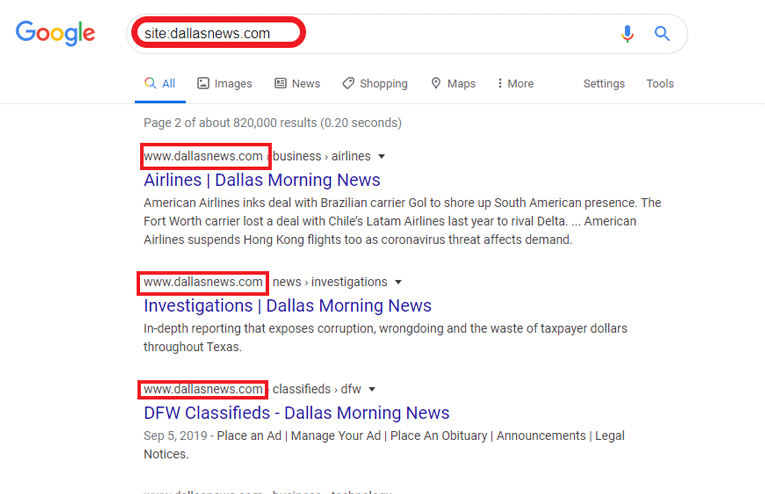This image appears to be a screenshot from a Google search results page. The Google logo, located at the top left, features its characteristic letters in the following colors from left to right: blue, red, yellow, blue, green, and red. To the right of the logo is the prominently displayed search bar. Inside the search bar, on the far left, the search query "site:dallasnews.com" is visible. On the far right within the search bar, there are two icons: a microphone icon followed by a magnifying glass icon.

A red border highlights the search query "site:dallasnews.com." Directly below the search bar are several navigation categories labeled from left to right as: All, Images, News, Shopping, Maps, More, Settings, and Tools. Further down, the text indicates that this is page two of approximately 820,000 results, which were generated in 0.20 seconds.

The middle of the image displays three distinct search results. The first result is a link to "www.dallasnews.com," specifically under the Business Airlines section. The second result links to a News Investigations page on "dallasnews.com." The third result points to the Classifieds and DFW section on the same site.